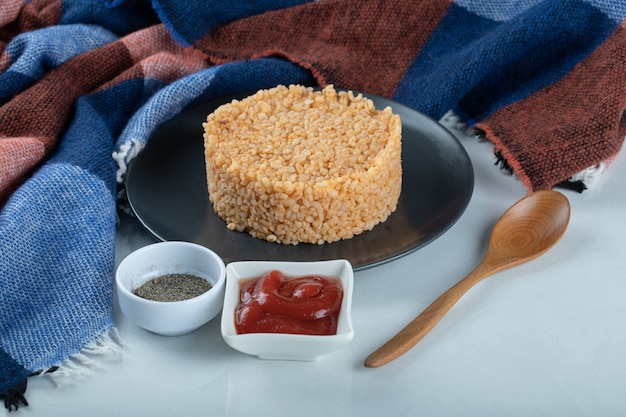The image depicts a round, cylindrical rice cake or Rice Krispie treat, light brown in color with whiter grains, placed on a black plate atop a white table. The table is partly covered by a plaid blanket with a checkered pattern in light blue, dark blue, light brownish-red, and dark brownish-red colors, draped around the dish. Alongside the main dish, there is a wooden spoon positioned at a 45-degree angle, with its scooping part facing the upper right. To the right of the black plate is a small square white bowl filled with ketchup. Nearby is a smaller round white bowl containing a black substance, likely pepper or some kind of spice. The overall setting suggests a cozy, homey atmosphere.